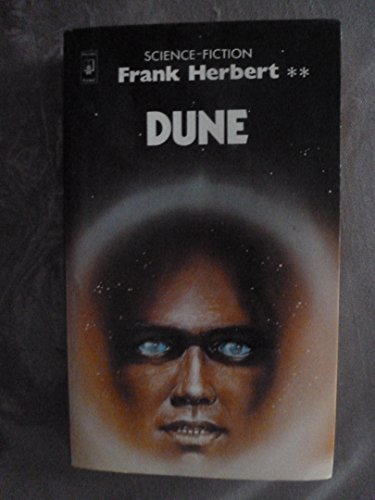The image depicts the cover of a book titled "Dune" by Frank Herbert, classified as science fiction. The top of the cover features the text "SCIENCE FICTION" in bold, all-capital white letters. Beneath this are the author's name, "Frank Herbert," presented in bold font but not in all capitals, flanked by two asterisk signs. The title "DUNE" is prominently displayed below his name in large, all-capital white letters.

The central image on the cover is a hauntingly eerie face with an open mouth displaying rows of white teeth. The face is tan in color, complemented by strikingly large, light blue eyes encircled by black rings, giving an impression of being glazed over. The figure seems to have dark black hair. Surrounding the face is a circular white emanation, contrasting against the predominantly black background of the entire cover. An additional small, indistinguishable white logo is positioned at the very top left corner of the cover. The image of the cover is set against a gray background, possibly on a table or against a wall, though the exact setting is not clearly defined.